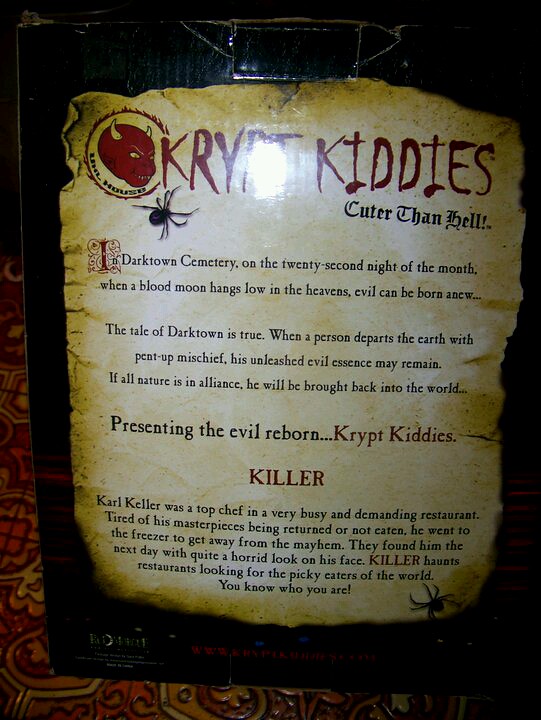This detailed image showcases a weathered, yellowish parchment paper with burnt and jagged edges. At the top, in striking red font, it reads "Crypt Kitties," accompanied by a devilish, dragon-like face on the right and a black spider beneath it. Directly below, the text says "Cuter than Hell!" In the main body of the parchment, an eerie tale unfolds: "In Darktown Cemetery on the 22nd night of the month, when a blood moon hangs low in the heavens, evil can be born anew. The tale of Darktown is true when a person departs the earth with pent-up mischief, his unleashed evil essence may remain. If all nature is in alliance, he will be brought back into the world." The narrative continues with the words, "Presenting the evil reborn… Crypt Kitties." Centrally placed below this is the word "KILLER" in bold black text, followed by a chilling paragraph: "Carl Keller was a top chef in a very busy and demanding restaurant. Tired of his masterpieces being returned or not eaten, he went to the freezer to get away from the mayhem. They found him the next day with quite a horrid look on his face. The killer haunts restaurants looking for the picky eaters of the world. You know who you are." Another black spider can be found at the bottom, adding to the haunting aesthetic.